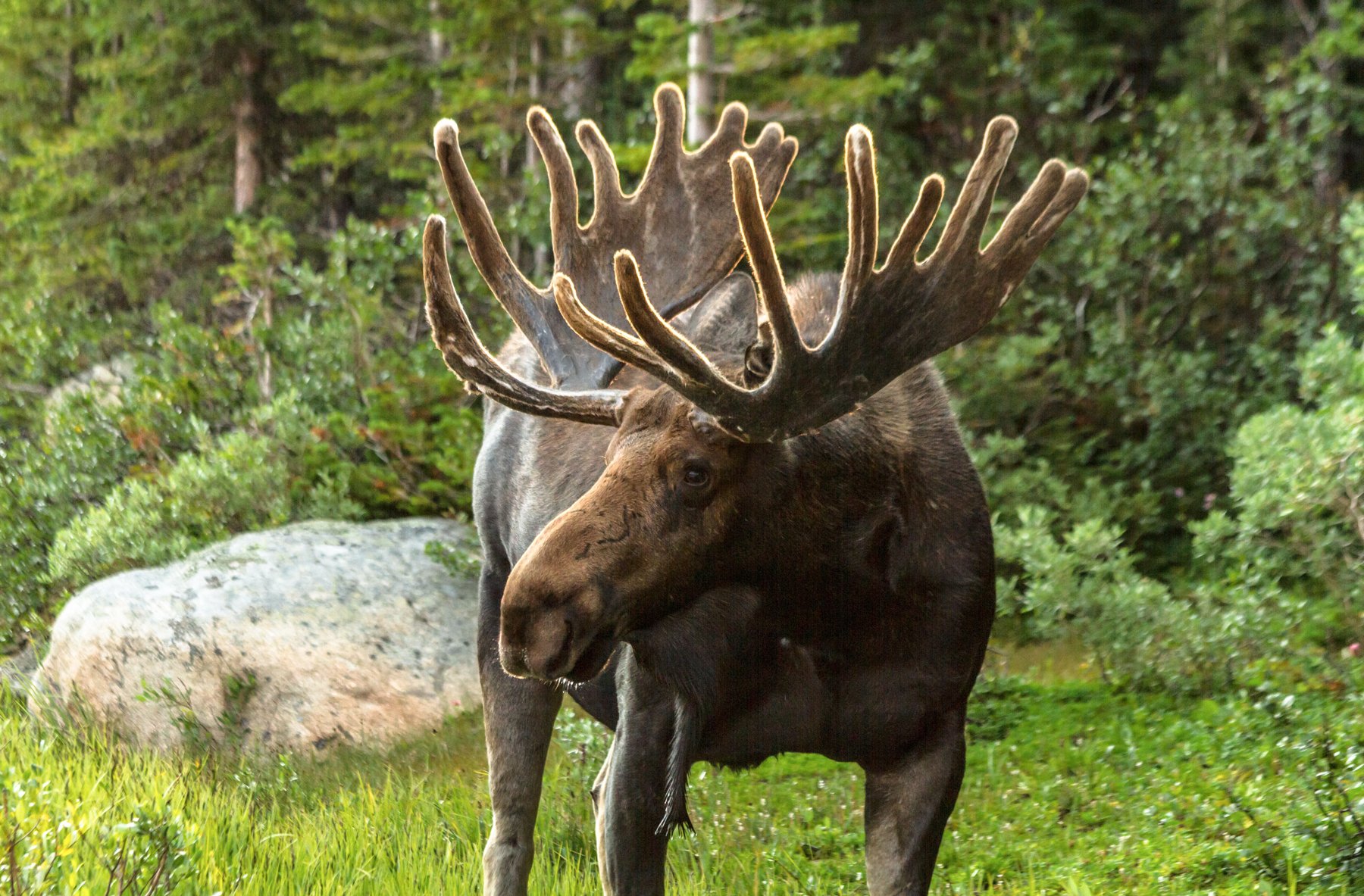This photograph captures a close-up of a fully grown, extremely large brown moose standing in a grassy open area of a lush, northeastern forest. Its head is turned slightly to the right, giving us a profile view and a full display of its large, brown antlers. The moose's mouth is closed, and its expression is neutral as it gazes into the distance. Notably, only one ear is visible. Dangling from its front right leg is a piece of fur or rope. To the left of the moose, a large gray boulder can be seen. Behind the moose is a very thick tree line composed of indigenous trees, contributing to the verdant and dense forest backdrop. There is also a white post directly behind the moose, though it's unclear whether it is a birch tree or something else.